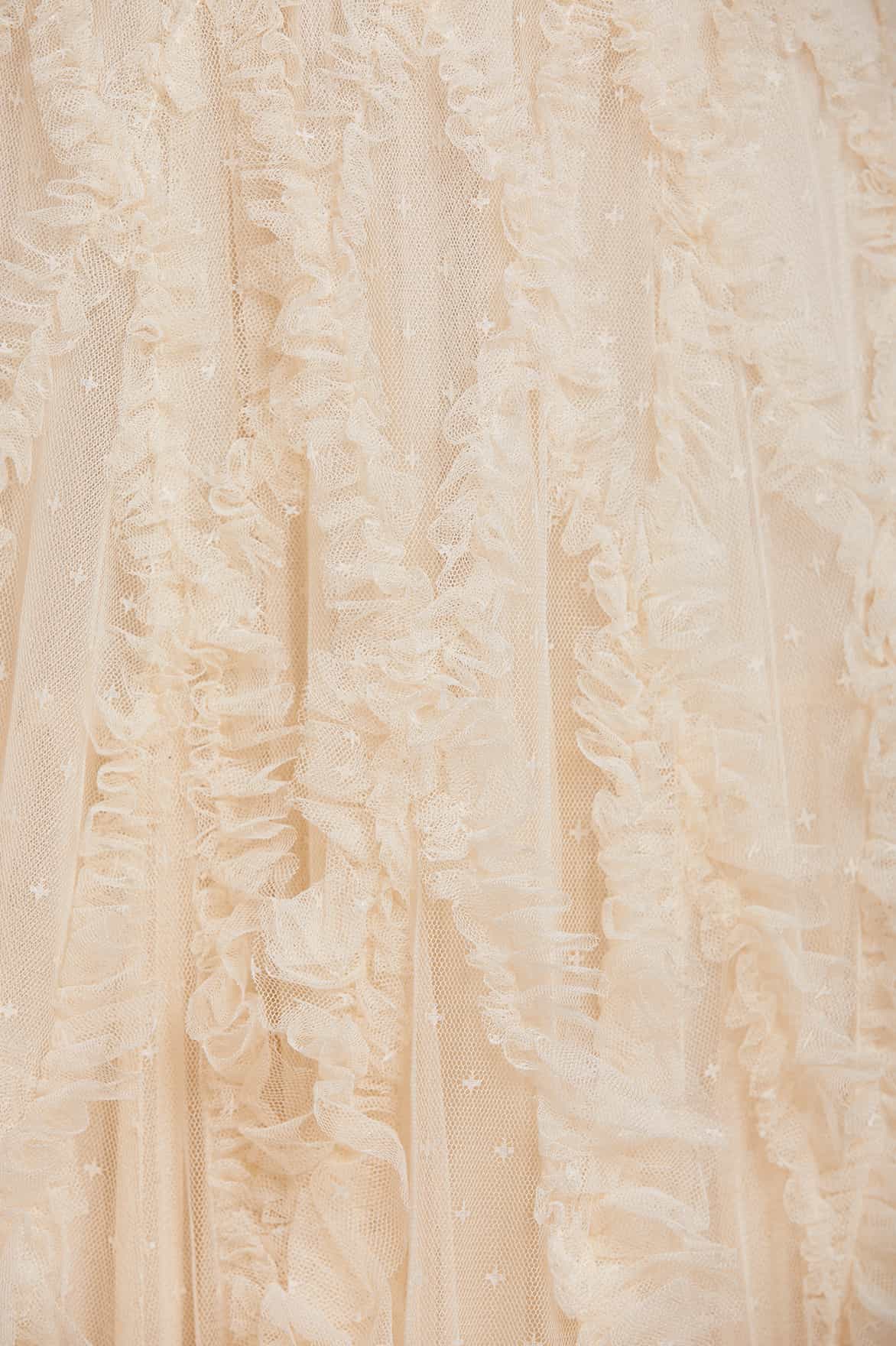This rectangular photograph captures a close-up view of a light pink fabric that completely fills the frame. The fabric features a distinctive design composed of vertical ruffled lines, creating an intricate texture reminiscent of tree bark with ravines and ridges. These ruffled lines form multiple puffs and intersect to make "X" shapes throughout the fabric. Overlaid on the light pink base, there appears to be a delicate lace sheet adorned with small, light cream-colored plus signs or stars, adding a subtle decorative element. The detailed texture and intricate patterns on the fabric give it an almost otherworldly appearance, blending naturalistic and textile elements.